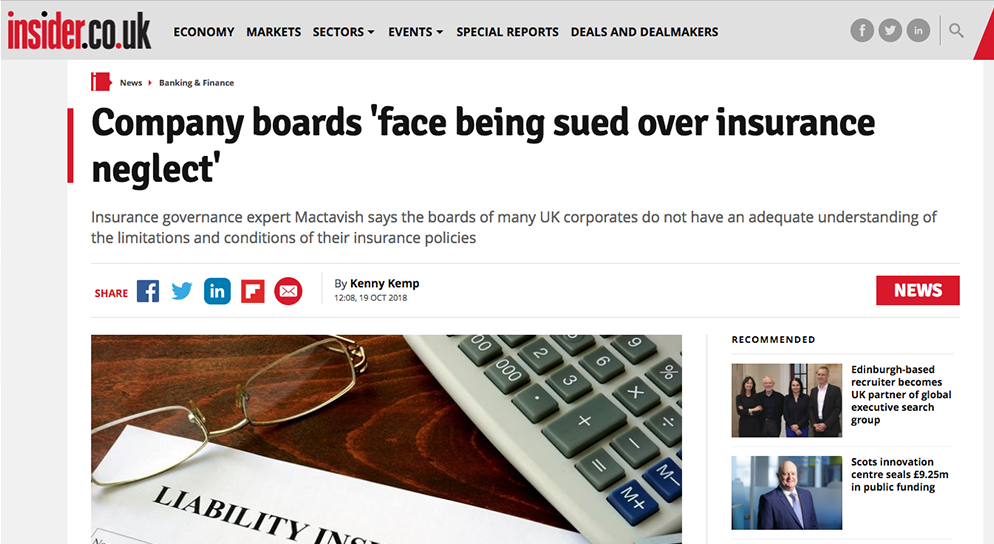This image captures a screenshot of a financial news website's homepage. At the top left, there is a red "Insider" label, followed by a black dot, "CO" in black, another red dot, and "UK" in black, forming the publication's branding. 

A horizontal menu spans across the top, featuring categories like "ECONOMY," "MARKETS," and "SECTORS," each with drop-down arrows for further options, followed by "EVENTS," "SPECIAL REPORTS," "DEALS," and "DEALMAKERS" in capital letters. 

On the right side of the menu, three small circles feature icons: "F" for Facebook, "R" for Twitter, and "IN" for LinkedIn, along with a gray magnifying glass icon for search functionality.

Below the navigation bar, the main content begins with a headline: "Company Boards Face Being Sued Over Insurance Neglect." The accompanying summary quotes Insurance Governance Expert MacDevish, highlighting the boards of many UK corporations' inadequate understanding of their insurance policies' limitations and conditions.

Further down, an illustrative graphic displays a desk with a piece of paper, a pair of glasses, and a calculator, reinforcing the topic of financial governance. Below this graphic are additional news highlights, including:

- "Recommended: Edinburgh-based recruiter becomes UK partner of global executive search group."
- "Scott's Innovation Centre seals £9.25 million in public funding."